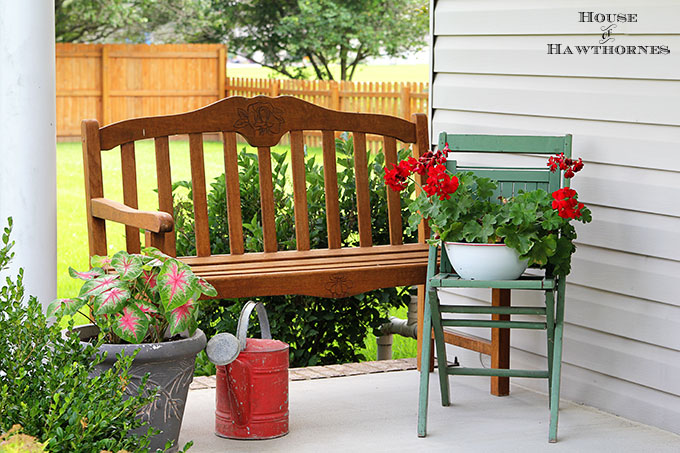This color photograph, in landscape orientation, captures a serene front porch scene of a house with gray horizontal siding and black text in the upper right corner reading "House of Hawthorns." Prominently featured is a wooden bench located at the end of the porch between a white column on the left and the house on the right. In front of the bench is a small folding chair, painted a light grayish-green, holding a white ceramic planter dish with vibrant red begonias and green leaves.

To the left foreground of the porch, there is a vintage red watering can with a silver handle and spout, showing signs of wear. Next to it is a tall gray planter with a philodendron plant that has green leaves with pink centers. The porch overlooks a yard filled with green grass and flanked by shrubs. Enclosing the yard is a wooden fence that is taller and light-colored on the left side and shorter on the right, with dark green trees providing a natural backdrop. The photograph exemplifies representational realism, offering detailed depiction and balance of the outdoor space.